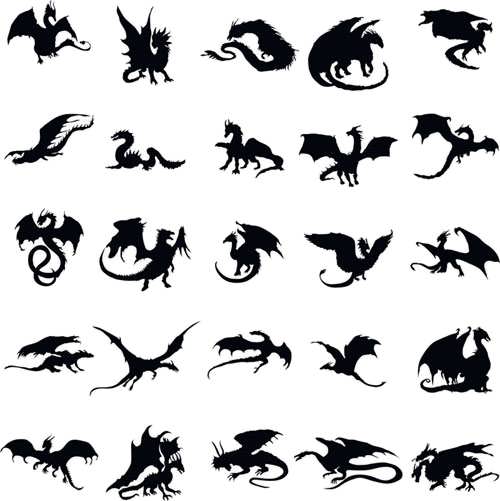This photograph features a grid of 25 distinct black dragon silhouettes, arranged in a precise 5x5 formation against a stark white background. Each dragon design is unique, showcasing an array of styles from traditional European dragons to more elongated, lizard-like forms. Notable variations include a two-headed dragon in the bottom right corner and a serpentine dragon on the left of the middle row. The silhouettes are ink-like and icon-sized, equally spaced, with some dragons depicted mid-flight with wings spread wide, while others have their wings folded. The composition emphasizes the diverse and imaginative representations of dragon forms, efficiently rendered in a minimalist yet striking style.